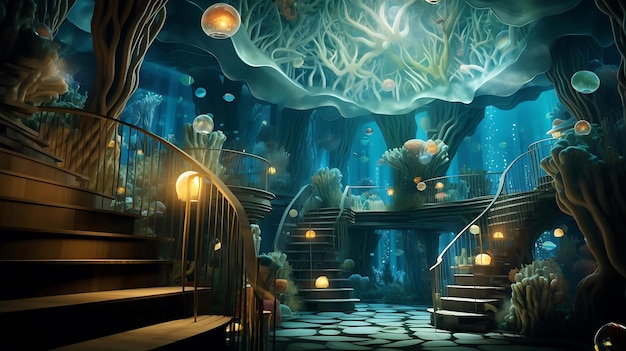This detailed image depicts an enchanted, fantasy-themed room characterized by an aquatic ambiance. The room features three distinct staircases—one on the left, one on the right, and one in the middle—each adorned with lighted globes. The space is draped in a blue-tinted light, adding to its otherworldly atmosphere. Tree trunks rise majestically from the ground to the ceiling, where an arrangement of white, connected lines and floating, branch-like aquatic objects are suspended. The ceiling also hosts various hanging lanterns, casting a mysterious glow. Among the details are fish swimming in the background, contributing to the aquatic theme, and scattered greenery, including cacti and other plants. The overall environment is dark and somewhat cavernous, with a ground that appears charred or cracked, amplifying the room's magical and mystical feel.